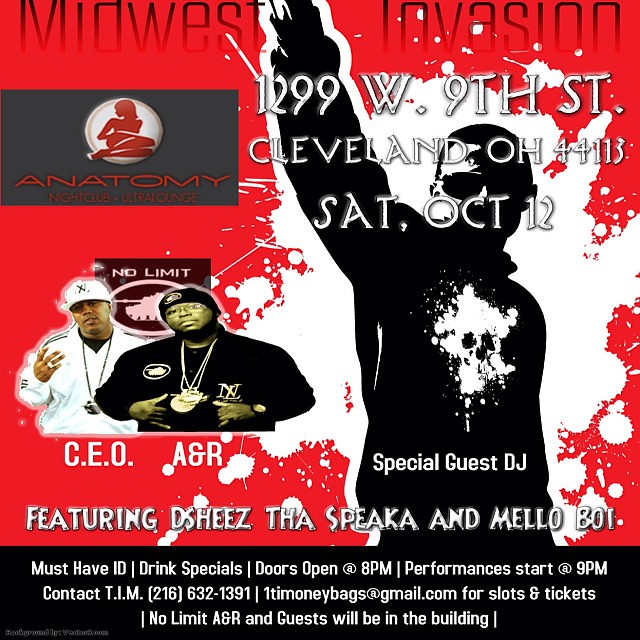This advertisement is for a live music event called "Midwest Invasion" at Anatomy Nightclub Ultra Lounge, located at 1299 West 9th Street, Cleveland, Ohio 44113, on Saturday, October 12th. The primary colors are red and white with black and white text. Prominently displayed in the top left corner is the Anatomy Nightclub logo featuring a red silhouetted woman lounging provocatively. Below this, a photograph of two performers, CEO and A&R, standing in front of a logo that reads "No Limit," is shown. On the right side, there's a shadowy black and white image of a man with his arm raised, which complements the announcement of a Special Guest DJ. The event will feature performances by Deshies, The Spica, and Mellow Boy. Important details include: "Must Have ID," "Drink Specials," "Doors Open at 8 p.m.," "Performances Start at 9 p.m." Additionally, contact information provided features a phone number, T.I.M. at 216-632-1391, and an email, 1timoneybags@gmail.com, for slots and tickets. Attendance by No Limit, A&R, and guests is highlighted at the bottom of the flyer.